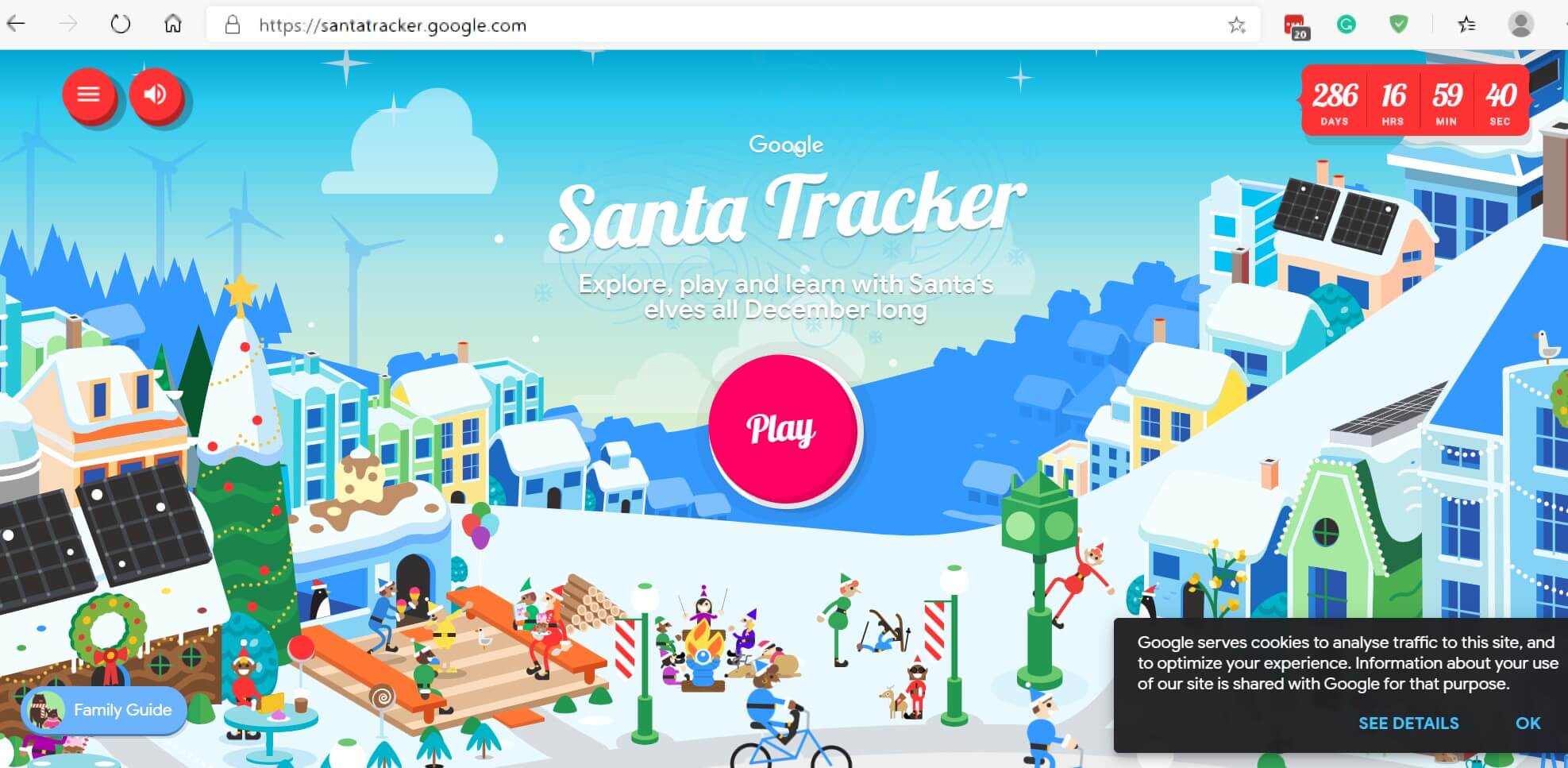The image depicts a screenshot of the homepage of the website "https://santatracker.google.com" displayed on a computer monitor. The top portion of the screen features a light gray navigation bar. On the left side of this bar, there are three icons: a left-pointing arrow (highlighted), a right-pointing arrow (not highlighted), and a nearly circular icon with an arrow. Next to these is a home symbol. Centered in this top section is a search bar prefaced by a lock icon, indicating a secure connection. Adjacent to the search bar is a star icon for bookmarking. Further to the right, there are four additional icons, and at the far right, there is a circle containing a silhouette of a digital person.

Below the navigation bar is a digital art section, featuring a nighttime sky with stars transitioning into a lighter blue with clouds. Dominating the middle of this section is text that reads: "Google Santa Tracker - Explore, Play, Add, and Learn with Santa and Elves all December long." Below this text is a round magenta button labeled "Play."

The visual background resembles a town or cityscape with various buildings, some of which have large solar panels. Wind turbines are visible in the background, accentuating the eco-friendly theme. Trees and gently rolling hills contribute to the scenery. The scene is bustling with activity: elves (mistaken initially for children) are seen riding bikes, climbing light poles, and engaging in various tasks. There is a particular building where elves are seated on benches, adding to the lively atmosphere.

At the bottom right of the screen, there is a horizontal rectangular black area that contains information about Google's use of cookies, along with options to "See Details" or "OK." In the bottom left of the screen, there is an oval-shaped blue area labeled "Family Guide."